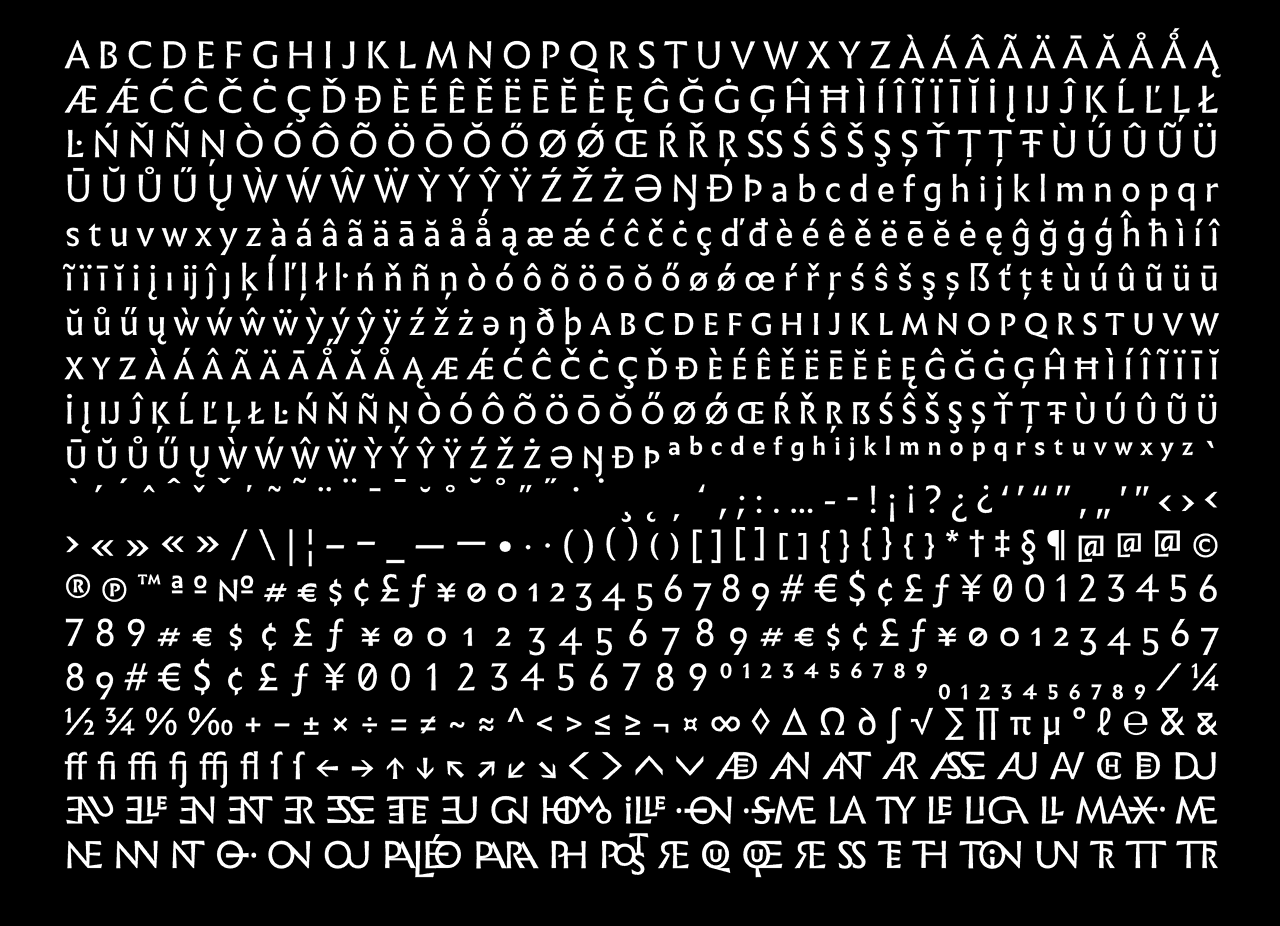This image, likely sourced from a tablet or desktop, showcases a comprehensive keyboard character map within a large black box. The array, rendered in white font, includes an extensive collection of characters ranging from the standard English alphabet, in both lowercase and uppercase, to various letters equipped with diacritical marks. Additionally, it features special symbols, punctuation marks, hyperscripts, and subscripts. Among the assortment are Cyrillic and Spanish language letters, as well as mathematical operators like the not equal sign, percentages, and division symbols. The bottom section displays numerous currency symbols, including those for pounds, euros, dollars, cents, francs, and yen, alongside trademark, copyright, and registered symbols. Furthermore, the collection comprises several Greek alphabet characters, including pi, and possibly other unfamiliar symbols. This illustrative compilation also includes estimation symbols, greater than and less than signs, plus or minus, and other diverse mathematical and typographical symbols.